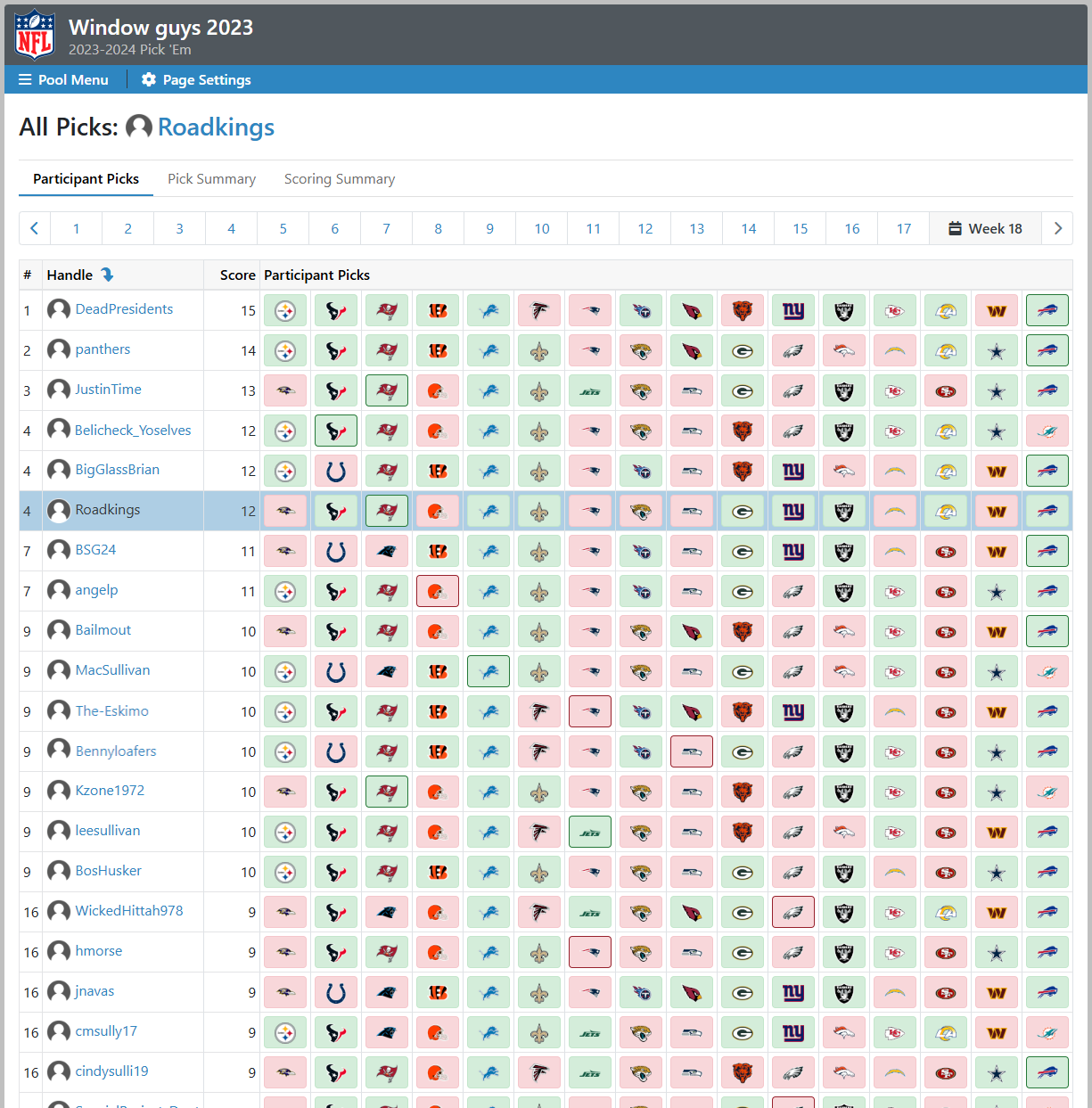The image features a detailed selection interface on a white background. At the top, the heading "All Picks" is displayed prominently, flanked by a left arrow on one side and a right arrow on the other, adjacent to an indicator for "Week 18" which includes a small calendar icon. Below this, there are two tabs labeled "Participant Picks" and "Pick Summary".

A blue box near the middle contains a hashtag and handle, accompanied by a downward-pointing arrow. Below that are the terms "Score Participant Picks" and "Tie", although the latter is partially cut off. 

The main table lists participants with various details. The first participant is labeled "Old School" and has the tag "Score Participant Picks: 11" along with a series of pink and blue icons, and a tie score of 46. 

"Josh Allen's Mustache" is highlighted in blue, showing "11 picks" and a tie score of 55.5. The other participants listed include "Mack", "Cosmo", "OEG", "Otto Wattriff", "Smirnoff Ice Hole", "Billy Mack", "A-Hole", "Millsy", "N-Mack", "Crid", "Birdman", "Loader", and "Chief". Each name is accompanied by a mix of pink and blue icons, each followed by respective numbers.